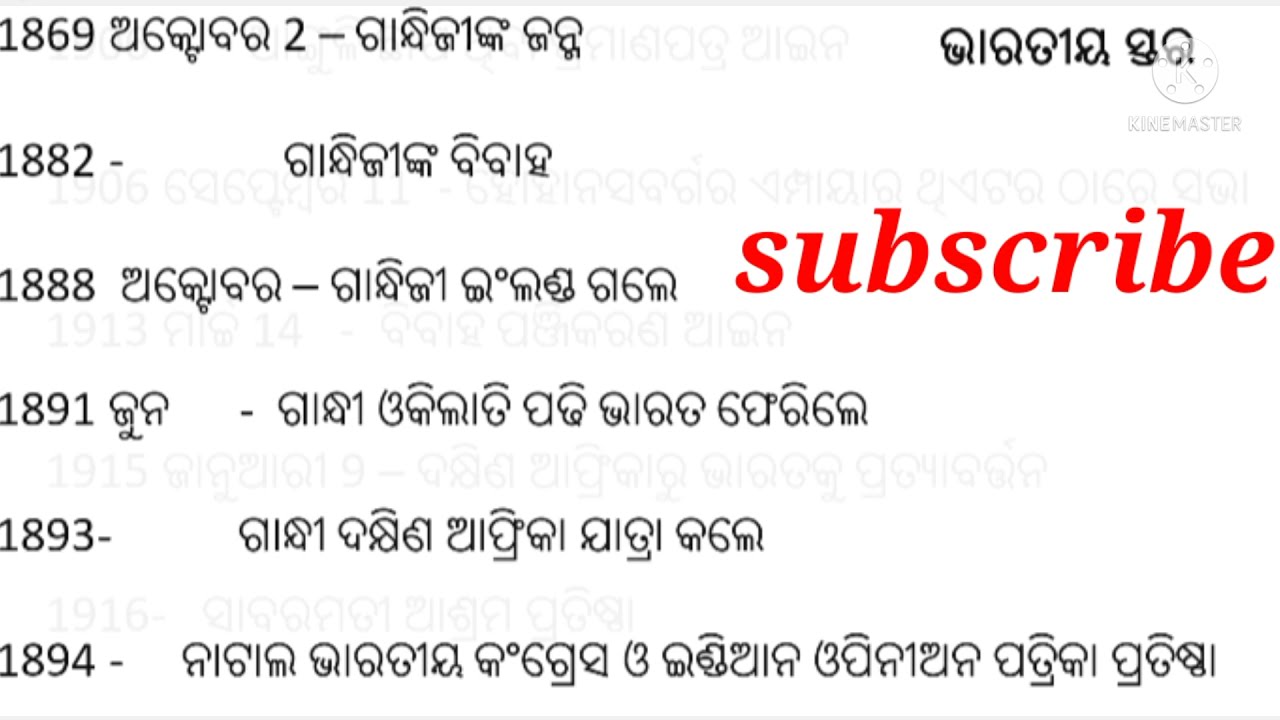The image depicts a minimalistic design with a predominantly white background and various lines of black text. Each line begins with a year, specifically 1869, 1882, 1888, 1891, 1893, and 1894. To the right of each year is a line of characters in an unidentified foreign language, possibly resembling computer code. On the far right side of the image, about a third of the way down, the word "subscribe" appears prominently in red text. The overall layout features a transparent aesthetic, enhancing its sleek, website-like appearance.